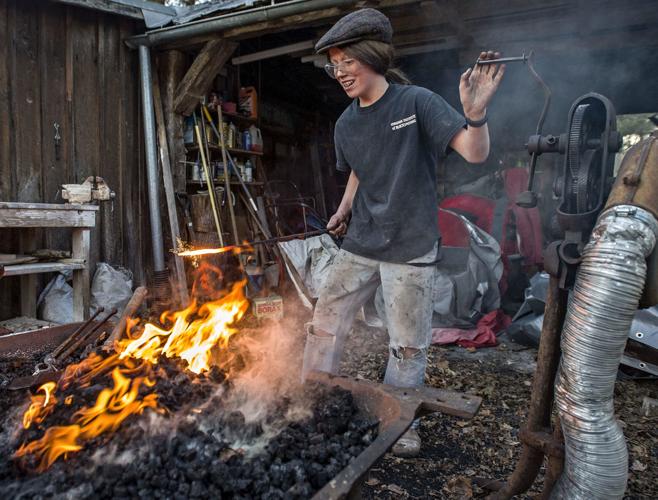A detailed color photograph captures a woman engaged in blacksmithing outside beside a disorganized shed. She is wearing torn and dirty whitish blue jeans, a black t-shirt, and a gray cap, possibly a beret or a Scully cap. Her long brown hair is tied back, and she wears clear safety glasses over what appear to be braces. The woman is holding a long iron poker with its red-hot, fiery tip in her right hand, indicating she has been heating it in a fire pit filled with glowing orange flames and black coals. With her left hand, she operates a hand crank attached to a cylindrical mechanism likely providing air to intensify the fire. The shed in the background is cluttered with tools, jars, bottles of paint and cleaners, a metal tube resembling a dryer vent, and various other items. A wooden table stands to the left of the woman, contributing to the chaotic ambiance of the workspace. Despite the grime and intensity of her craft, the woman smiles, clearly immersed in her blacksmithing activity.